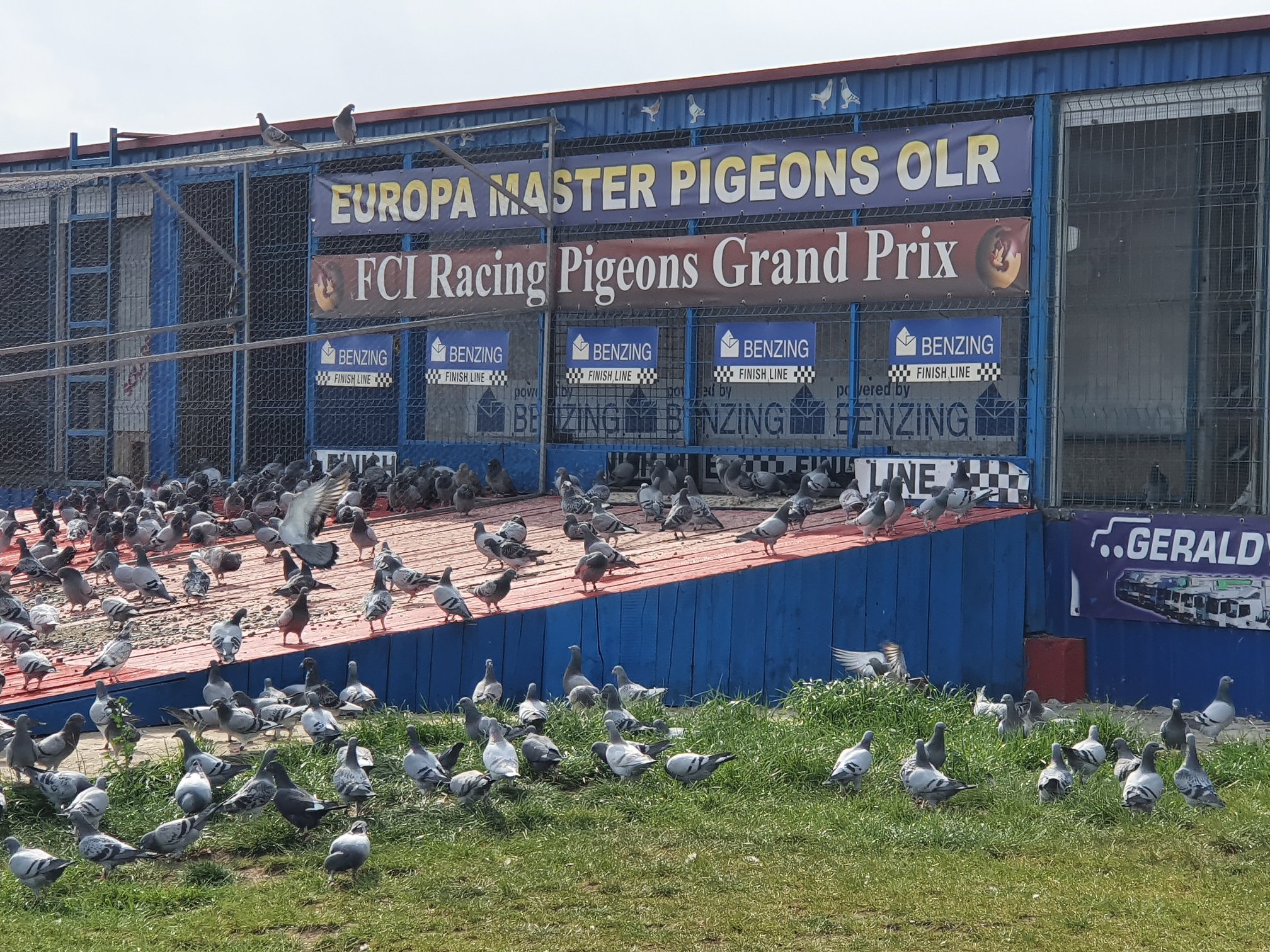In this detailed image description, we see a large congregation of pigeons at a blue building that is part of a pigeon racing event. The building, which is painted blue and features caged windows, serves as the starting point for the race. Prominently displayed are banners stating "Europa Master Pigeons OLR" and "FCI Racing Pigeons Grand Prix," alongside another sign, "Benzing Finish Line." Some of the pigeons are enclosed within the cage-like structure attached to the building, while others freely explore the surrounding area. A distinctive red ramp with blue underskirting extends from the building, covered in what appears to be scattered seed, attracting the birds. The setting includes green grass in the foreground and gives the impression of hundreds of pigeons either pecking at the food on the ramp or resting on the grass. There are no people visible in the scene, highlighting the sheer number of pigeons gathered for the race at this remarkable blue structure.